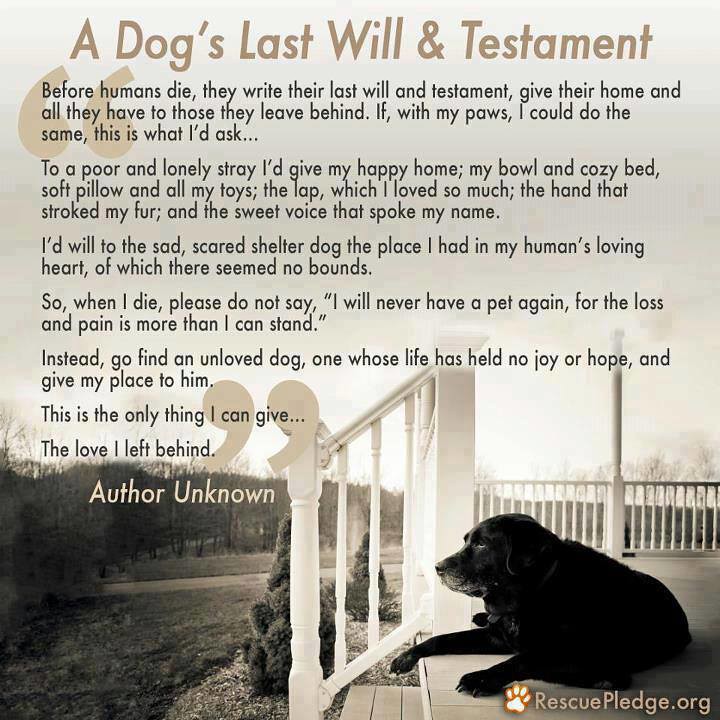The image is a sepia-toned, square photograph that serves as an advertisement titled, "A Dog's Last Will and Testament". It features a lengthy and poignant quote printed over the photo, which narrates a dog's imagined testament, expressing its wishes for its belongings and love to be given to a lonely stray dog. The quote is displayed in light brown and black fonts. In the bottom right corner of the image, there is a solemn black dog sitting on a porch with a white fence, staring out at a lawn with large trees on a cloudy day. The dog's expression and the lack of vibrant colors amplify the melancholic mood of the scene. In the same corner, the name of the organization, Rescue Pledge, along with a paw print, is also shown, indicating support for pet adoption.